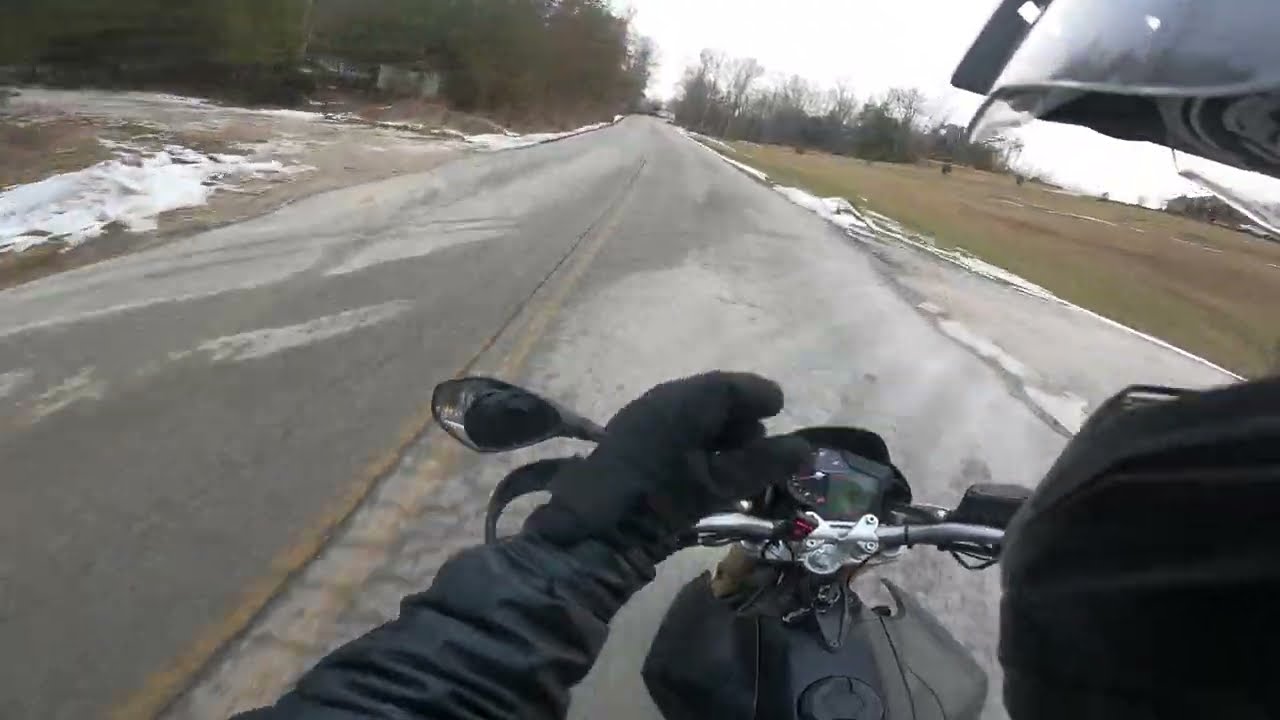The image captures a first-person perspective of someone riding a motorcycle down an old, two-lane road made of worn grayish concrete. You can see the rider’s left hand, clad in a black glove, gripping the silver handlebar. A heavy jacket sleeve and some wiring for the brakes are visible as well. The rider’s helmet, with a clear visor, is partially visible in the top right corner of the picture. The road is bordered by patchy snow on both sides, with the left side having more noticeable snow and some dark bare ground, while the right side features mostly brownish, grassy areas. Bare trees line both sides of the road, with a white, possibly run-down house partially hidden among the trees on the left. The background is filled with blurry bare trees and some buildings peeking through. The overall scene suggests a cold, late winter ride.